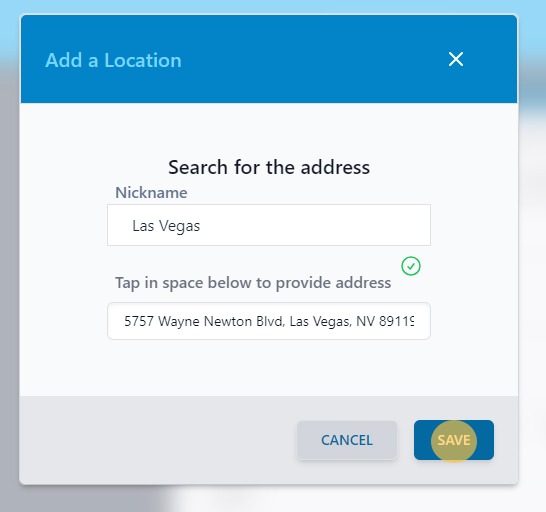This image depicts a vibrant and user-friendly website interface. At the top, a light blue horizontal bar spans the width of the page, extending slightly downward on both the left and right edges. Nested within this bar is a slightly darker blue strip that prominently features the text "Add a Location" in blue, with a white 'X' icon on the far right side for closing the section. Directly below, there is a light gray rectangular box that contains a black text field labeled "Search for the address." Below this, there's an entry labeled "Nickname" accompanied by a text box filled with the name "Las Vegas."

Beneath these elements, a prompt reads "Tap in space below to provide address," inviting user interaction. Slightly above and to the right, a green circle with a checkmark signifies confirmation or success. Further down, a white box displays the indicated address for the location being searched.

At the bottom of the interface, a horizontal light gray strip stretches across the page, incorporating a gray "Cancel" button and a blue "Save" button. The "Save" button is particularly prominent, featuring a rounded green corner with the word "Save" in white text.

The overall design is framed with color variations: the light blue at the top and darker gray on the left side, transitioning to light gray around the right edge and bottom. This cohesive color scheme aids in guiding the user's focus within the interface.